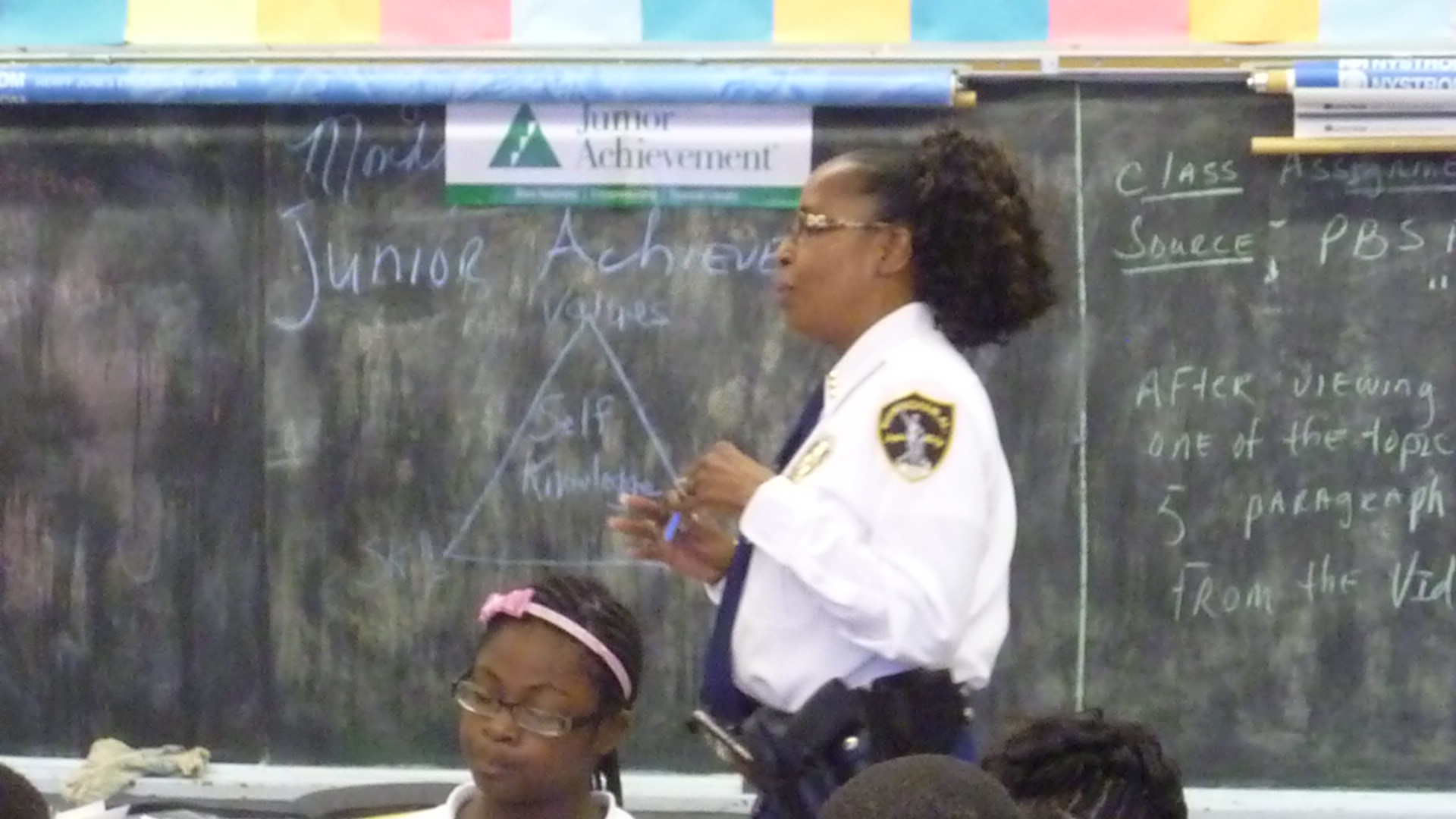The photograph captures an indoor classroom setting, with a well-used chalkboard spanning the entire length of the image. Central to the photo is an African-American police officer, a woman wearing glasses, a white shirt, and a dark blue tie. Her uniform also features a visible badge and shoulder patch, indicating her official capacity. She is slightly turned to the side, possibly holding a pen or piece of purple chalk, which matches the writing on the chalkboard behind her. The chalkboard is filled with various writings, including a prominently featured "Junior Achievement" program title, a triangle with "self-knowledge" inscribed inside, and a class assignment sourced from PBS, instructing students to write five paragraphs based on a video. At the top of the chalkboard, there is a thin banner and a colored border, adding to the classroom's educational ambiance. In front of the police officer, at the bottom of the frame, are several students seated at desks. Among them, a young girl with a pink bow in her hair and another student with glasses looking downward are visible. The scene is brightly illuminated, suggesting it’s taken during the day, emphasizing the active and engaged learning environment.